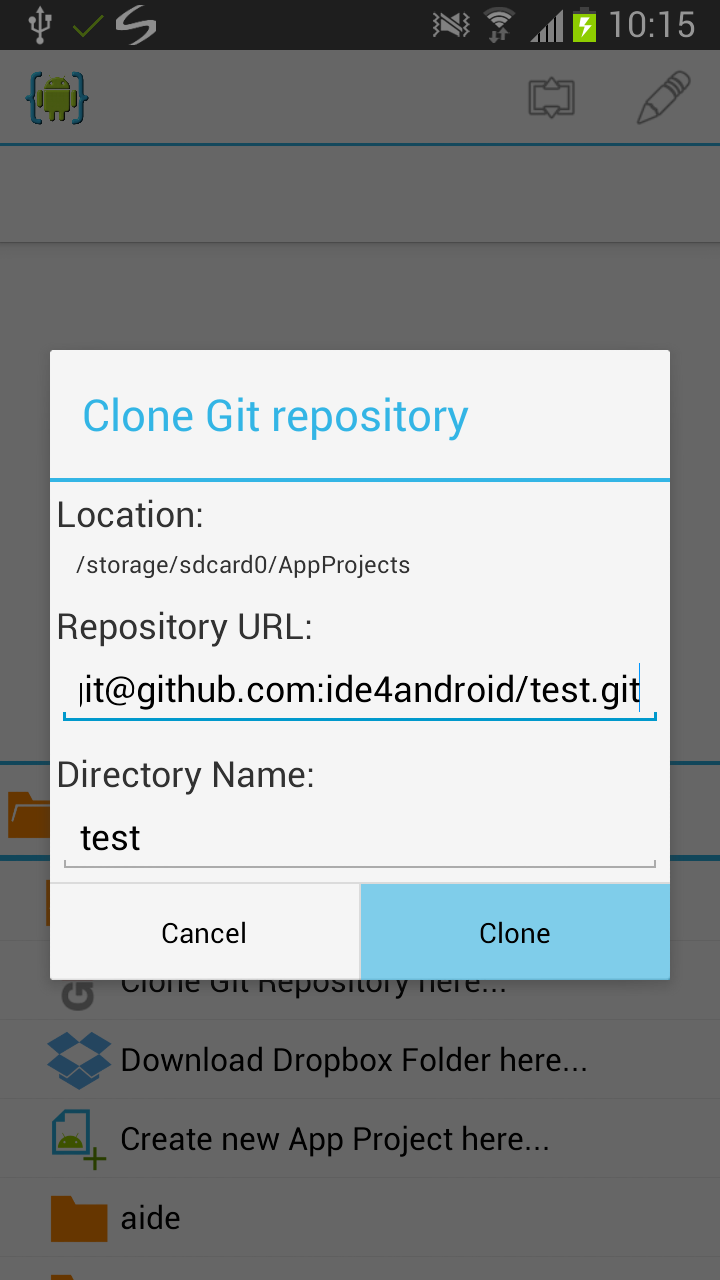The image displays a screenshot of a smartphone interface. In the upper left corner, there are several icons: the universal USB symbol, a check mark, an avatar, and a slanted 'S' logo. The screen indicates that the sound is turned off and there is an active connection. The battery status is shown to be full, and the time displayed is 10:15.

Additionally, in the upper left corner, there is a small robot avatar. Icons for navigation (up and down arrows) and an editing tool (pencil) are also visible. The background of the interface is dark gray, with lines separating different sections.

A pop-up window occupies a central area of the screen, with a slightly off-white background. The pop-up window is titled "Clone Git Repository," with the 'Git' acronym spelled out as "G-I-T." Within the pop-up, there are fields labeled "Location," "Repository URL," and "Directory Name." The location is specified as "storage/SD card0/app projects," and the Repository URL is "git@github.com:IDE-Android/test.git." The directory name is simply "test." At the bottom of the pop-up are two buttons: "Cancel" and "Clone," with "Clone" highlighted in blue.

In the dark gray background behind the pop-up, several buttons are partially visible, labeled "Clone Git repository here," "Download Dropbox folder here," "Create new app project here," and "AIDE," which is associated with a red folder icon. The detailed depiction suggests that the screenshot is taken from a developer tool interface on a smartphone.